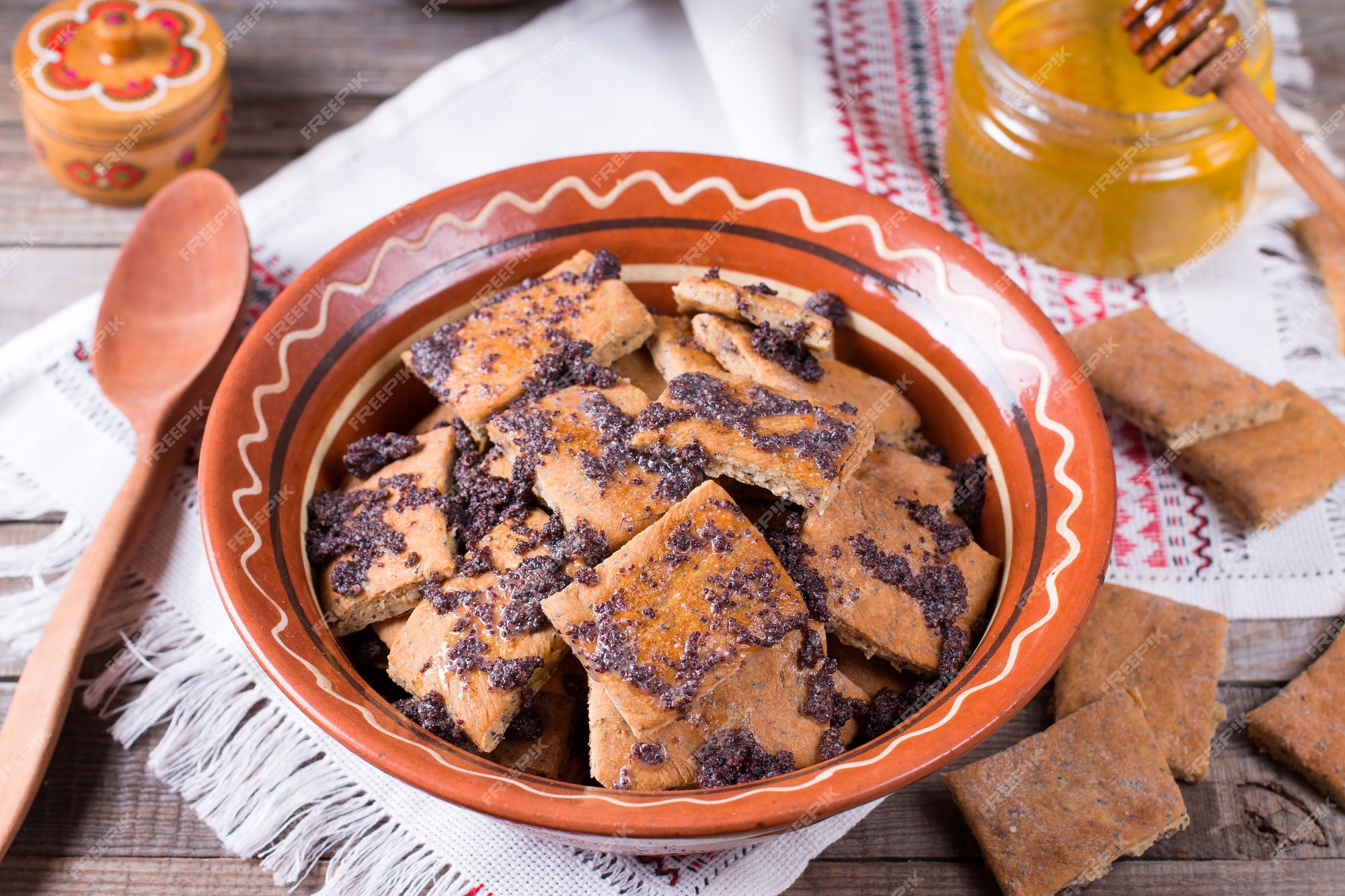A detailed color photograph depicts an orange bowl with intricate black and white wavy designs near the rim, set atop a white, fringed knitted cloth on a wooden table. Inside the bowl are what appear to be soft, brown-topped graham crackers or cookies, lightly dusted with a mysterious dark substance, possibly seeds or fine crumbs. To the left of the bowl, a large wooden spoon lies on the cloth, while an open jar of golden honey with a honey dipper sticking out is positioned at the upper right corner of the image. Scattered around and outside the bowl on the table are additional pieces of the crackers or cookies. To the upper left, a small, closed container with a red floral design, its contents hidden, completes the scene.